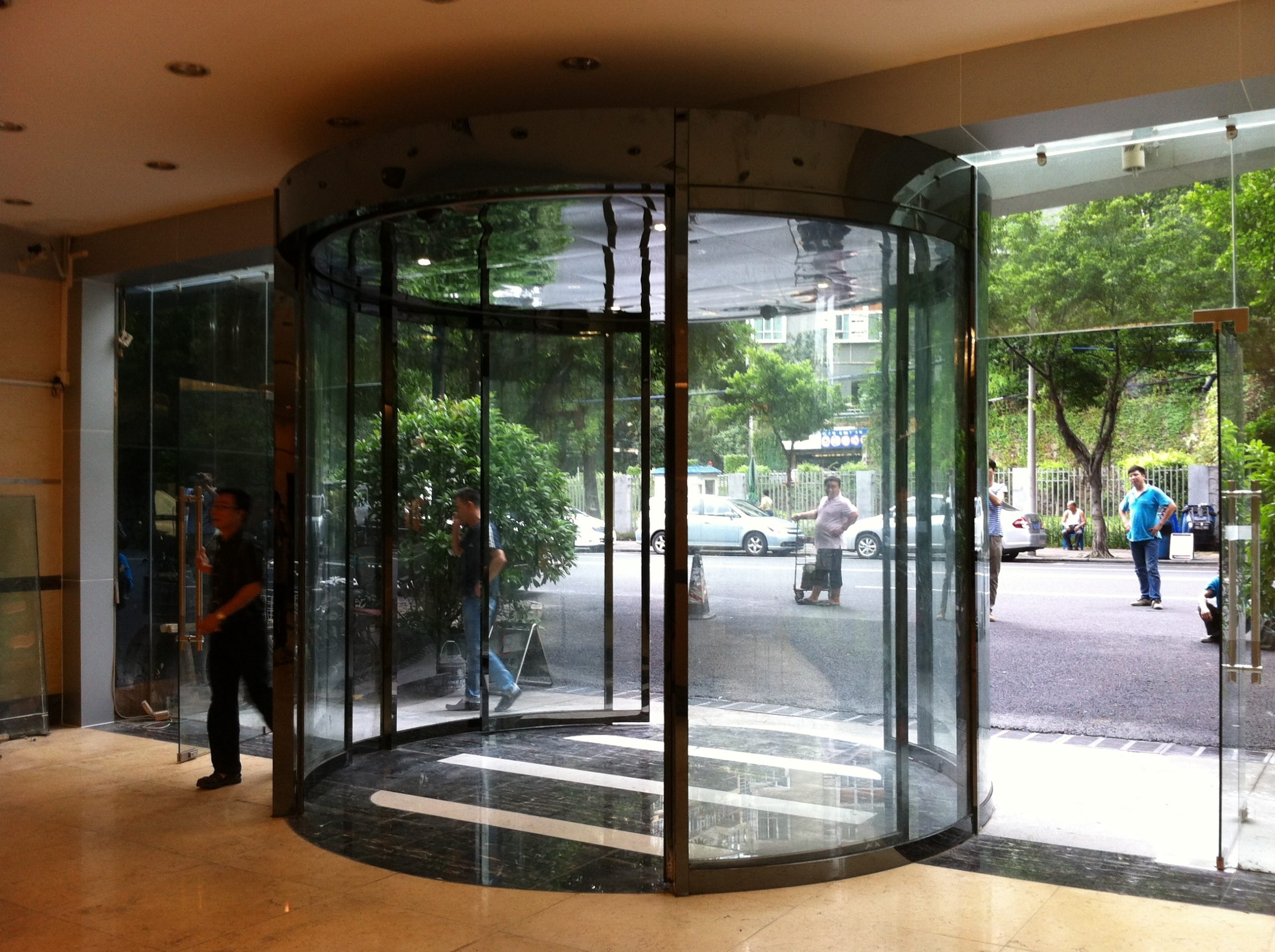The photograph captures the front entry of a building featuring a large cylindrical revolving door centrally positioned, flanked by single glass doors on either side with substantial metal handles. The entrance showcases a transition from black tiles within the revolving door to tan-colored tiles inside the building. The walls and ceiling inside are painted a whitish tan hue, complimented by multiple recessed light fixtures. Outside, the street is visible, covered with black asphalt and marked with white lines to indicate various traffic lanes. Several cars, mostly sedans, are parked along the sides of the road. The urban environment features people walking and standing near the entrance, some holding luggage or other items, with a couple of individuals engaged with cell phones. The exterior scene is complemented by green trees and shrubs, adding a touch of nature to the bustling city backdrop.